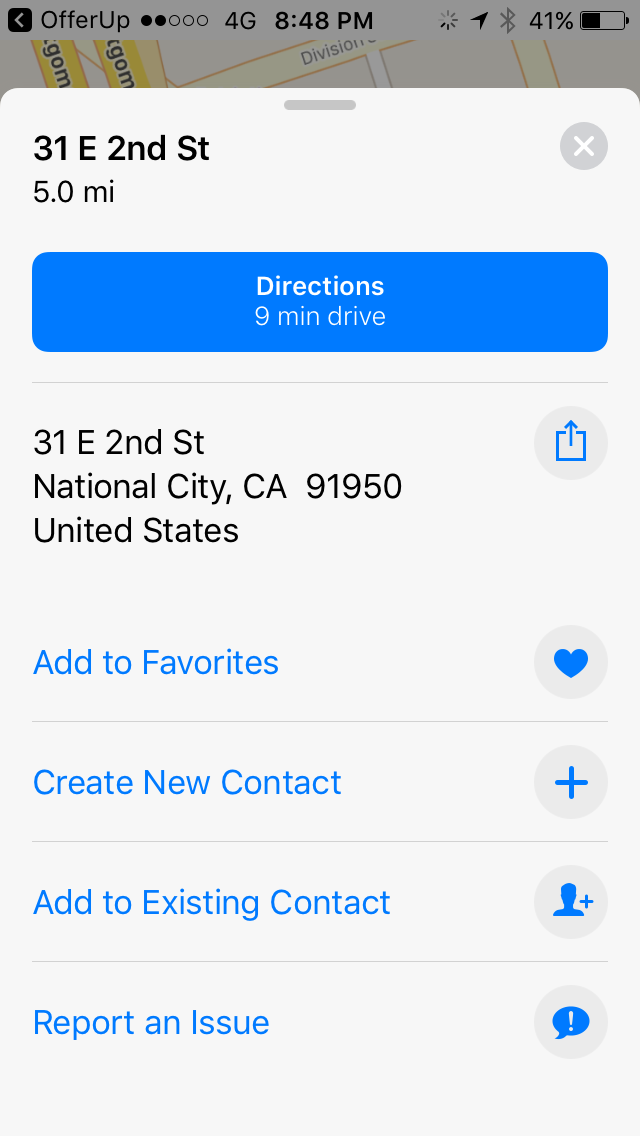This image is a screenshot captured on a cell phone. At the top of the screen, it displays "Offer Up" alongside various status indicators: 4G signal strength, Bluetooth icon, arrow icon, time (8:48 PM), and battery level at 41%.

The primary content of the screenshot is a pop-up displayed against a white background with minimal visible portions of a map underneath. The pop-up provides location details in various fonts and colors. The main text, written in black font, indicates the address "31 East 2nd Street" and the distance "5.0 MI." Beneath this, a blue box contains the text "Directions" in white font, specifying a "9 minute drive."

Further down, the address "31 East 2nd Street, National City, California, 91950, United States" is reiterated in black font. Following this, several interactive options are listed in blue font:
- "Add to Favorites" accompanied by a heart icon.
- "Create new contact" with a plus sign.
- "Add existing contact" alongside an illustration of a person's head and a plus sign.
- "Report an issue" with an exclamation mark inside a speech bubble.

There is a gray "X" in the corner of the white pop-up, indicating the option to close it.

The partially visible map behind the pop-up shows a white background with yellow streets and black font for place names. The pop-up obscures the majority of the map, leaving only the top portion visible.